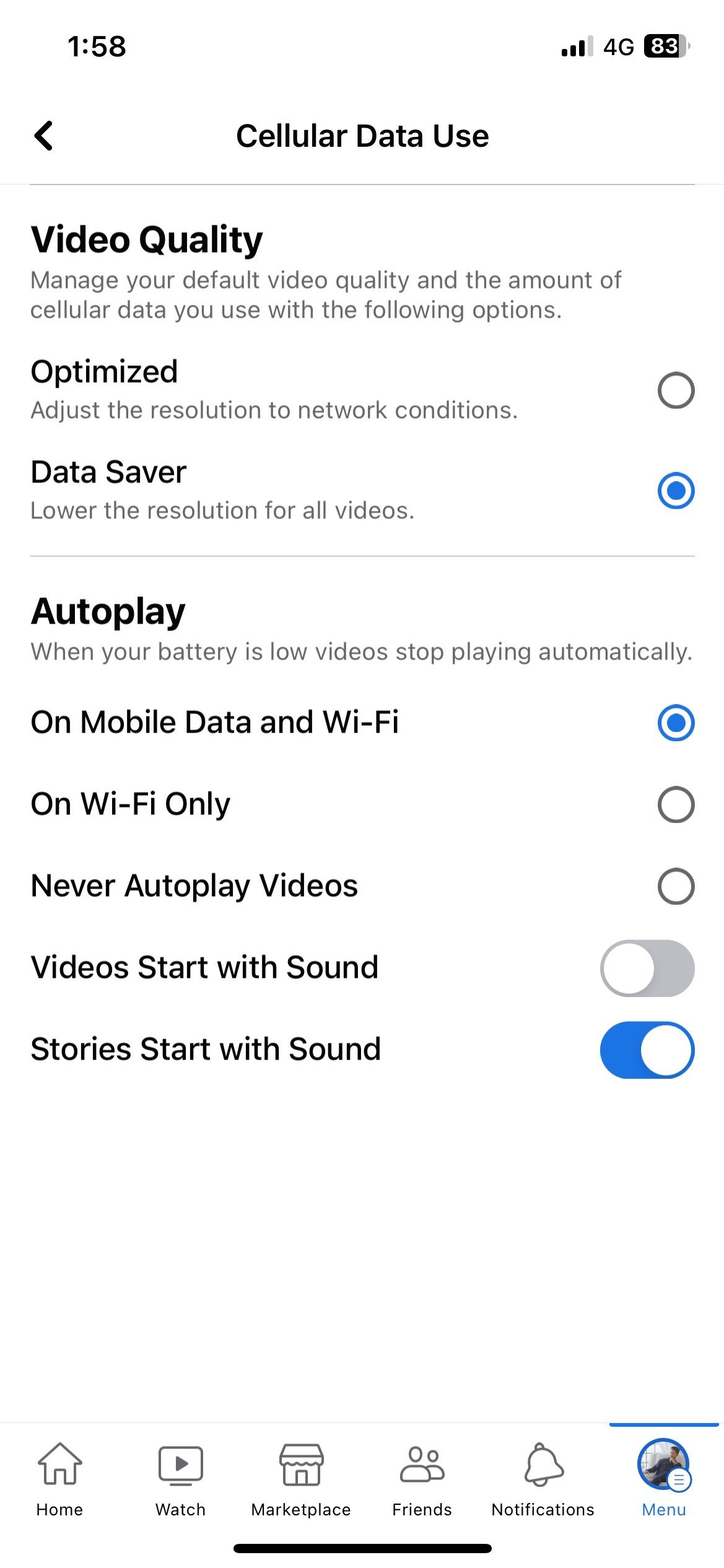This screenshot from a smartphone displays the cellular data usage settings, set against a white background. The time, shown at the top left corner, reads 1:58. To the top right, indicators display three out of four bars for signal strength, a 4G network connection, and 83% battery power.

At the top of the screen, centered text reads "Cellular Data Use," accompanied by a left-pointing arrow on the far left. Below this, in a boxed section separated by thin gray horizontal lines, the black text "Video Quality" stands out. It is followed by a smaller description in light gray: "Manage your default video quality and the amount of cellular data you use with the following options."

The options listed below include:
- "**Optimize**: Adjust the resolution to network conditions."
- "**Data Saver**: Lower the resolution for all videos." This setting is highlighted with a blue-filled circle on the right.

Further down, the section labeled "Autoplay" specifies different settings:
- "When your battery is low, videos stop playing automatically."
- "On mobile data and Wi-Fi," which is selected with a blue highlight.
- "On Wi-Fi only," indicating another option.
- "Never autoplay videos."

Additional settings include "Videos start with sound" and "Stories start with sound." The "Videos start with sound" option is unchecked, while "Stories start with sound" is highlighted.

At the very bottom of the screen, a horizontal black line separates the primary content from the navigation bar. This bar includes icons indicating Home, Watch, Marketplace, Friends, Notifications, and Menu. A profile photograph outlined in blue with a thin blue line horizontally above it is highlighted under the Menu section.